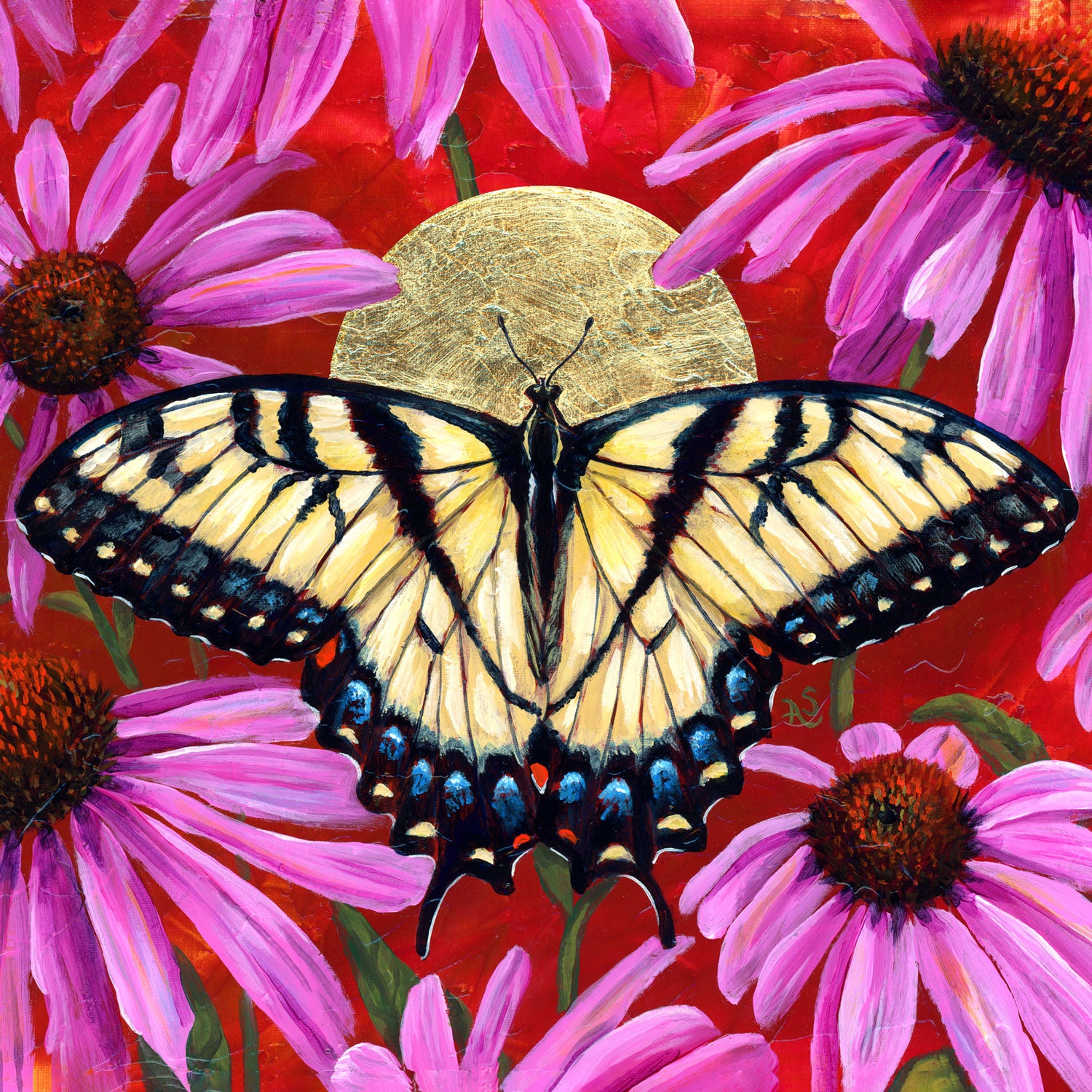This is a detailed painting of a stunning yellow butterfly, centrally positioned against a vibrant red background. The butterfly’s wings are fully spread, extending to the edges of the square-shaped image. Its wings are adorned with black ribbings and stripes, forming a distinctive V-shape pattern at their center. The butterfly features intricate blue dots at the tips of its wings, followed by yellow dots, all enclosed by a sharp black border. Its body, head, and antennae are black, giving it a striking contrast.

Behind the butterfly, there is an enigmatic round object, possibly a moon or a brass-colored disc, which highlights its head and antennae more clearly. Surrounding the butterfly are about six bright pink daisies, each showcasing around ten long petals with red, dandelion-like centers. The flowers are connected by green stems, adding a touch of greenery to the vivid scene. This composition beautifully captures the delicate and captivating essence of the butterfly amid the colorful floral and abstract elements.